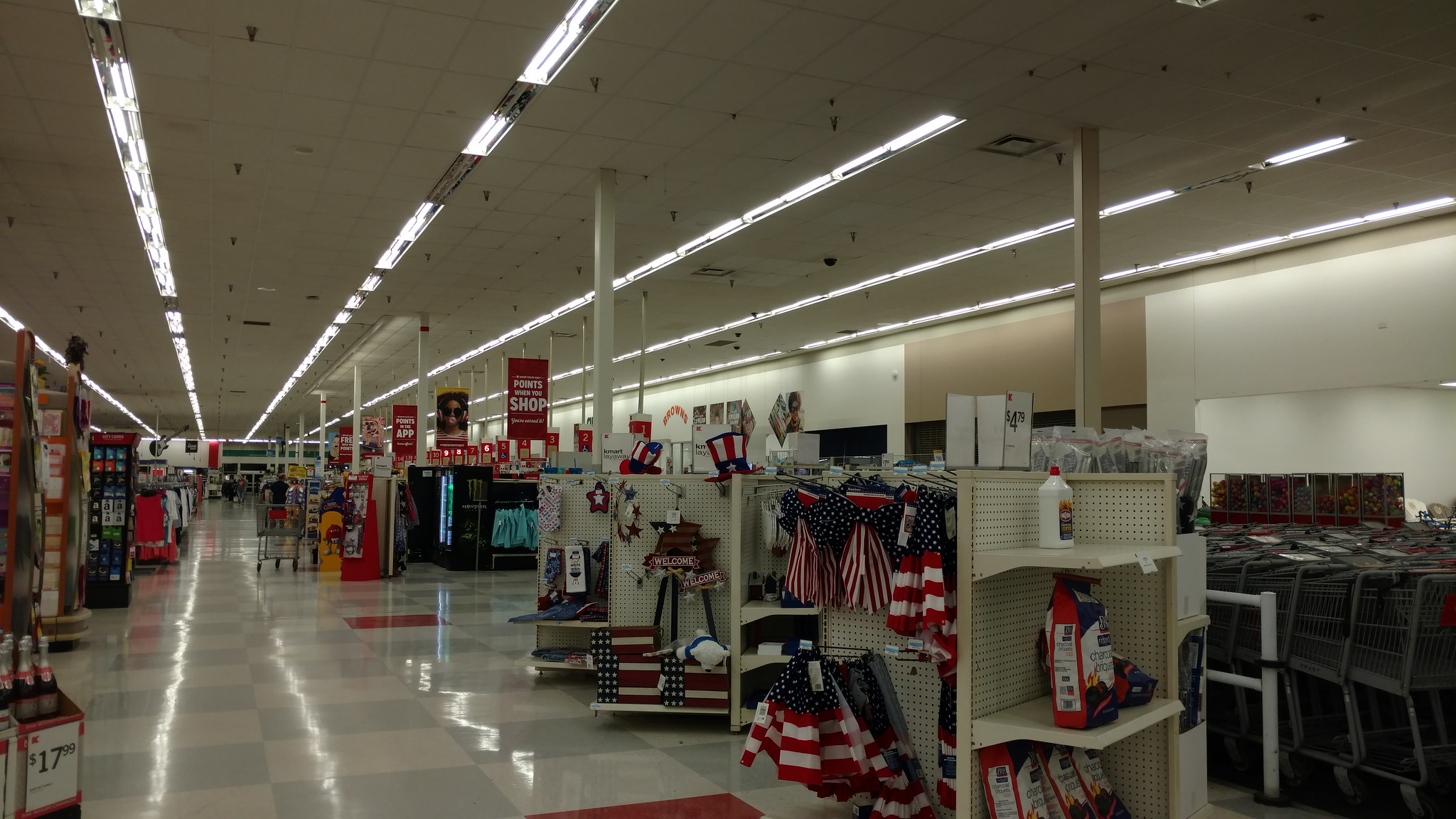This image captures the indoor view of a store, characterized by a long, narrow corridor lined with merchandise on both sides of an empty walkway extending into the distance. The store is illuminated by bright fluorescent lighting overhead. The floor is a shiny, reflective, gray checkerboard pattern. Multiple shelves and islands display various goods along the aisle. Nearest to the viewer, the shelves are stocked with barbecue grill supplies and a selection of red, white, and blue towels and other patriotic decor items. Further down the aisle, checkout lanes and additional food merchandise can be seen in the background.